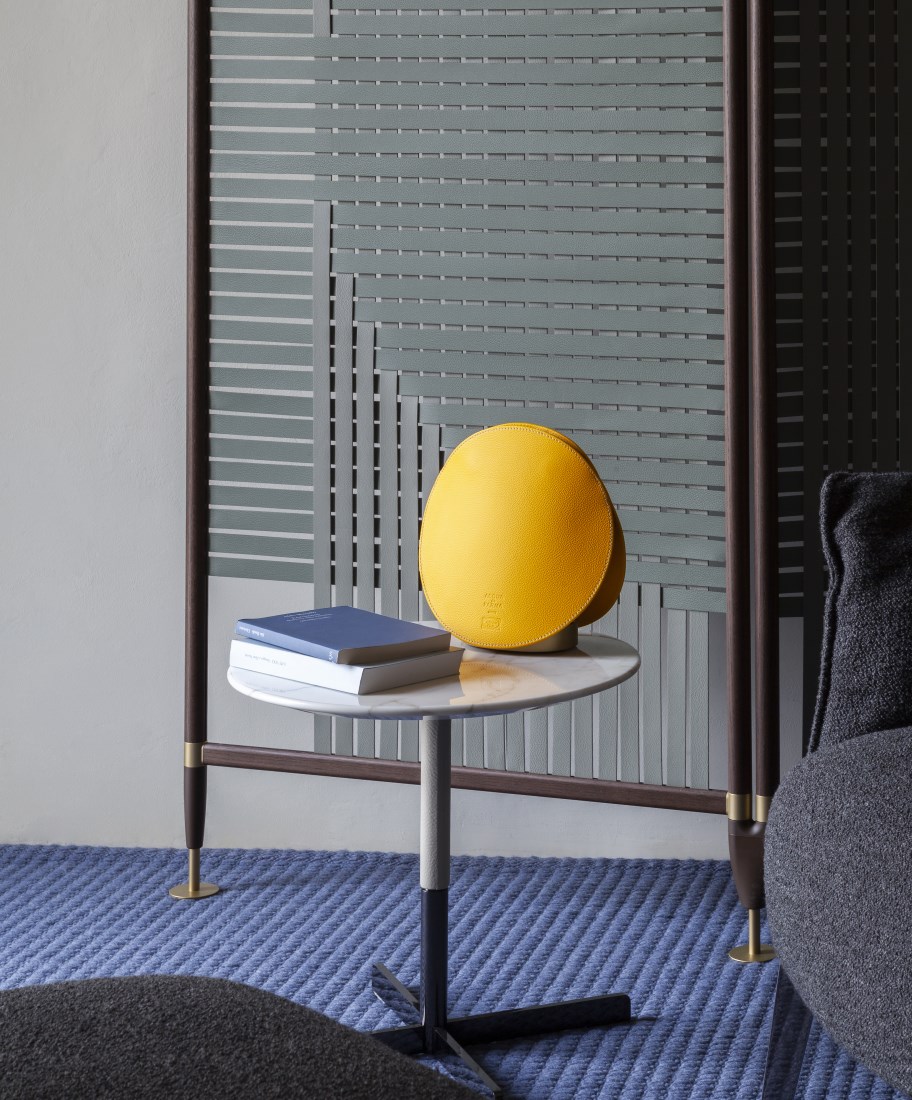This photograph captures a modern indoor scene featuring a round table with a light-colored, possibly marble, top and a thin cylindrical gray bar that transitions from a light gray at the top to a darker gray at the bottom. The table is supported by an X-shaped base. Resting on a blue, ridged carpet, the table holds two stacked books—one blue and the other white—and a circular yellow object, potentially a lamp or mirror in a leather case.

To the right, partially visible, is a gray chair with a cushion and backrest. In the background, there is a foldable, partition screen constructed with gray woven straps and framed in brown wood. The screen extends out of the image frame, and attached to its bottom are vertical strips and circular legs. The setting is minimalistic, with a gray wall enhancing the contemporary aesthetic.